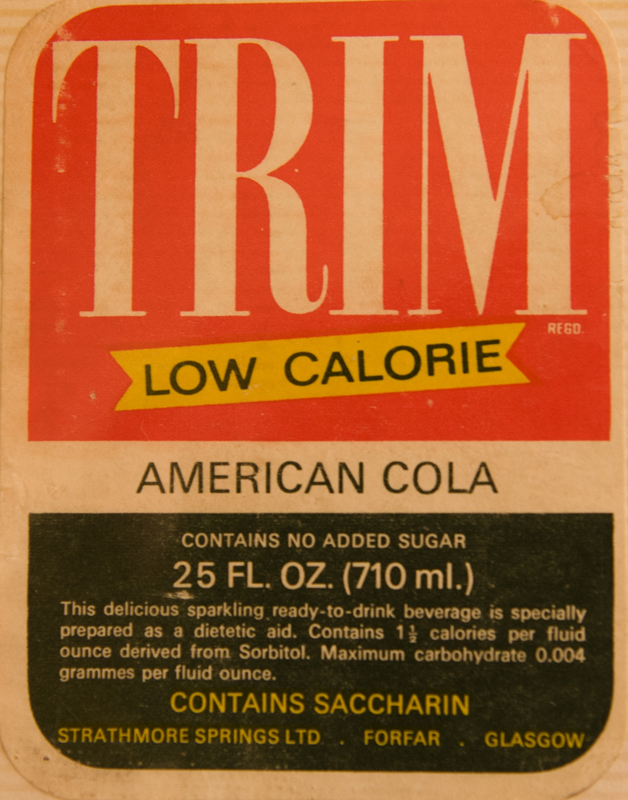This close-up photograph features a vintage label for Trim Low Calorie American Cola, showcasing its aged texture with faded colors and subtle dirt marks. The label, primarily in red, yellow, white, and black, prominently displays the word 'Trim' in tan letters on a red background at the top, with a yellow banner underneath bearing the words 'Low Calorie' in black. 'American Cola' is printed below in black letters, followed by details in tan on a black background at the bottom, stating 'Contains no added sugar, 25 fluid ounces, 710 milliliters.' The label also provides additional information: 'This delicious, sparkling, ready-to-drink beverage is specially prepared as a diet aid, containing one and a half calories per fluid ounce, derived from sorbitol, with a maximum carbohydrate content of 0.004 grams per fluid ounce. Contains saccharin.' The producer is identified as Strathmore Springs Ltd., located in Forfar, Glasgow.